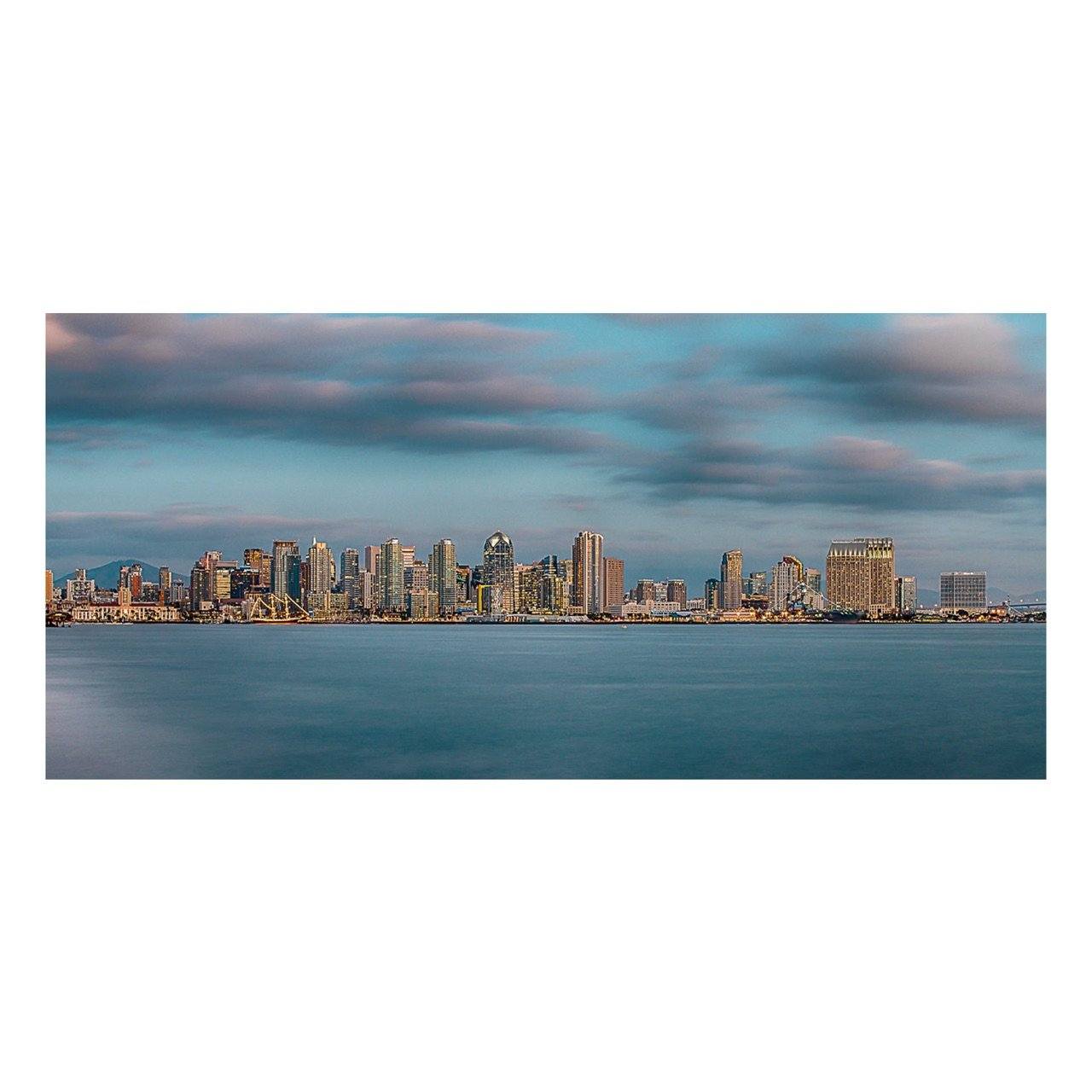This photograph captures a panoramic view of a city skyline seen across calm, dark blue waters, likely a river, small lake, or bay. The calm water of the foreground, devoid of waves, leads towards the expansive cityscape. The skyline features a diverse array of buildings, predominantly tall high-rises interspersed with shorter structures, indicating a bustling urban center. Close to the center, the buildings are densely packed, while they become more sparse towards both the left and right edges of the image. In the background to the left, a small mountain is faintly visible, adding a natural element to the urban scene. Overhead, the sky is adorned with a mix of grey and purplish clouds, some of which have stratus-like formations, all set against a deep blue sky. The lighting suggests the photo was taken during sunset, casting a soft, serene glow over the entire scene.